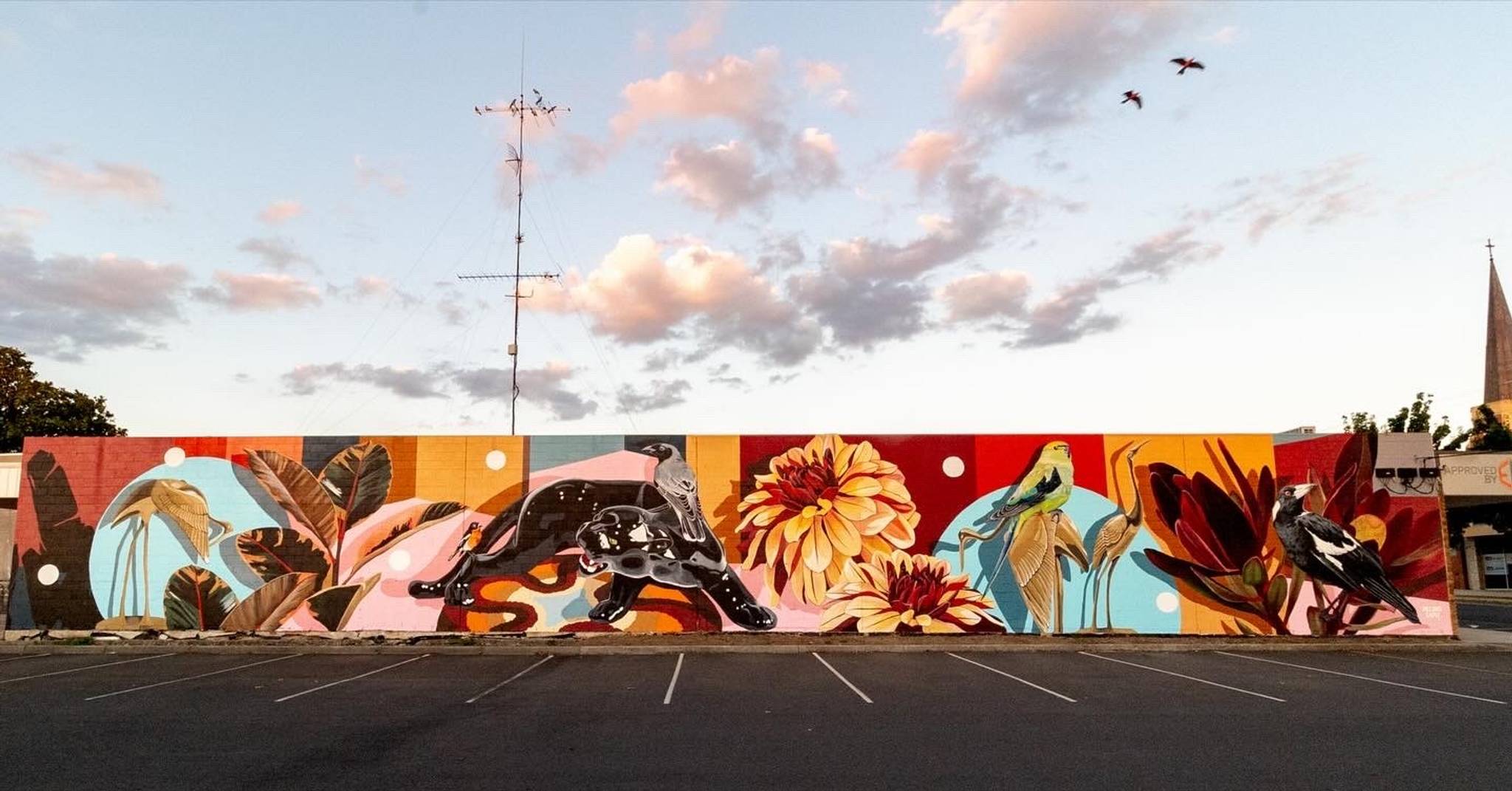The image captures a vibrant mural sprawling across a long wall, located in a parking lot devoid of cars. The scene is set against a daylight backdrop featuring a light blue sky scattered with dark grey and white clouds. The mural itself stretches approximately 100 feet horizontally and is brimming with a diverse array of vibrant and detailed illustrations. Vivid stripes in reds, yellows, blues, and oranges form the backdrop for an array of flora and fauna. 

Toward the left, the mural showcases a heron amidst palm-like leaves. As your eyes travel rightwards, you encounter an orange panther or cougar with a small bird perched on it. Further along, there's a large chrysanthemum-like flower, more leaves, and various birds. The mural is peppered with small white dots—four or five in total—whose significance is unclear.

In front of the mural, the parking lot features dark pavement with several white-lined spaces, suggesting a business-like area, possibly a strip mall. The mural, painted in warm tones of blues, greens, browns, and oranges, creates a striking contrast with the concrete surroundings, bringing a burst of nature and color to the urban setting.